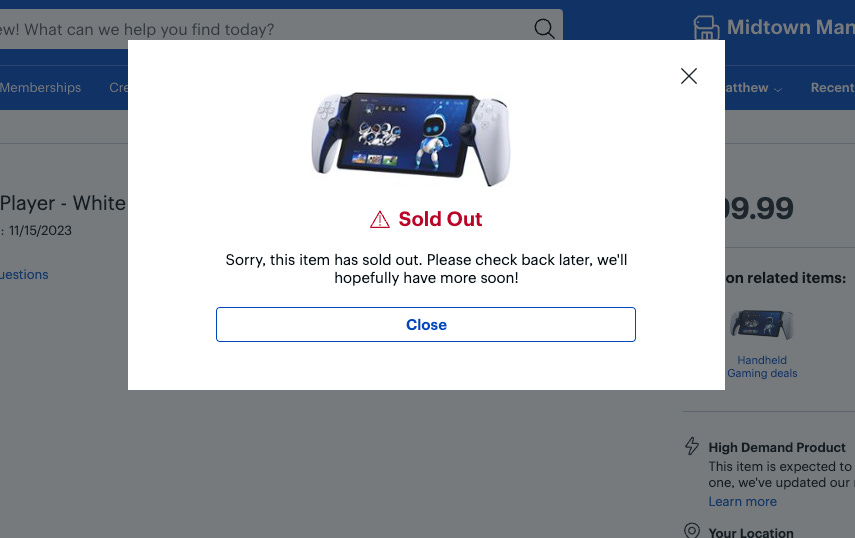This detailed caption describes a screen capture of a tech or business website, providing a comprehensive overview of its various elements and layout.

---

**Caption:**

The screen capture depicts a potentially tech-oriented or business website, characterized by multiple interactive elements and information sections. At the top, a grayed-out search box with text saying "What can we help you find today?" and a magnifying glass icon is prominently displayed. Below it, a blue business name and logo featuring a simplistic white building with a small price tag icon, partially reads "Midtown."

Further down, there are two white submenus; the first is labeled "Recent," and the second has a pop-up overlaying it. On the right side, the interface shows a section labeled "Memberships," with a partial view of a date entry stating "Player white 11-15-2023." There's also a blue link captioned "Questions."

Moving right again, there is a "Related Items" section in black text, highlighting a blue link titled "Handheld Gaming Deals," alongside another small black text entry indicating "High Demand Product" with a lightning bolt icon. The statement "This item is expected to" is cut off. Below, an announcement begins with "We've updated our," and further down, a prompt "Learn more" appears, followed by a location indicator with a pin icon and the text "Your location."

At the top of the image, a pop-up is visible, characterized by a white box with a gray "X" in the corner. Displayed within this pop-up is an image of a handheld gaming system in white, navy, and black, featuring two partial game controllers attached to a small tablet screen. The left controller showcases a directional pad, while the right has additional directional buttons and two round black buttons on either side. The tablet's screen displays a navy background with numerous white and blue robots piled together, alongside a more distinct white, blue, and black robot adorned with piercing blue eyes, a blue cape, and a small antenna.

At the bottom of this pop-up, red text states "Sold out," followed by the message in black text: "Sorry, this item has sold out. Please check back later. We'll hopefully have more soon." Lastly, a blue button labeled "Close" is prominently placed below the sold-out message.

---

This caption provides a detailed visual description of the entirety of the screen capture, allowing readers to get a full sense of the webpage's layout and content.